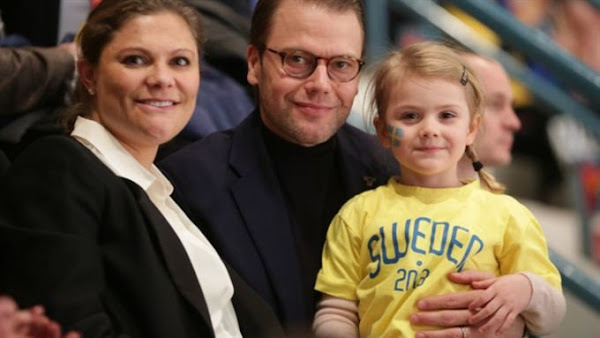In this vibrant photograph, we see a warmly dressed family of three, likely consisting of a mother, father, and their young daughter. The woman on the left, appearing to be in her early 40s, has brown hair neatly tied back and radiates a warm smile towards the camera. She is dressed in a sharp, black jacket over a white collared blouse. Standing beside her, in the center, is her husband. He sports short brown hair and brown-rimmed glasses, smiling with his lips together. He wears a black turtleneck under a dark blue sports jacket. On the right, their daughter with very blonde hair, parted to the side and styled in braid adorned with a black band and hair clip, sits happily. Her face is decorated with face paint, including a striking four-leaf clover on her cheek. She wears a cheerful yellow short-sleeved shirt with "Sweden" printed on it over a long-sleeved beige shirt. The background reveals a lively setting with several other people around, adding to the richness of the scene. The photograph is dated 2013.